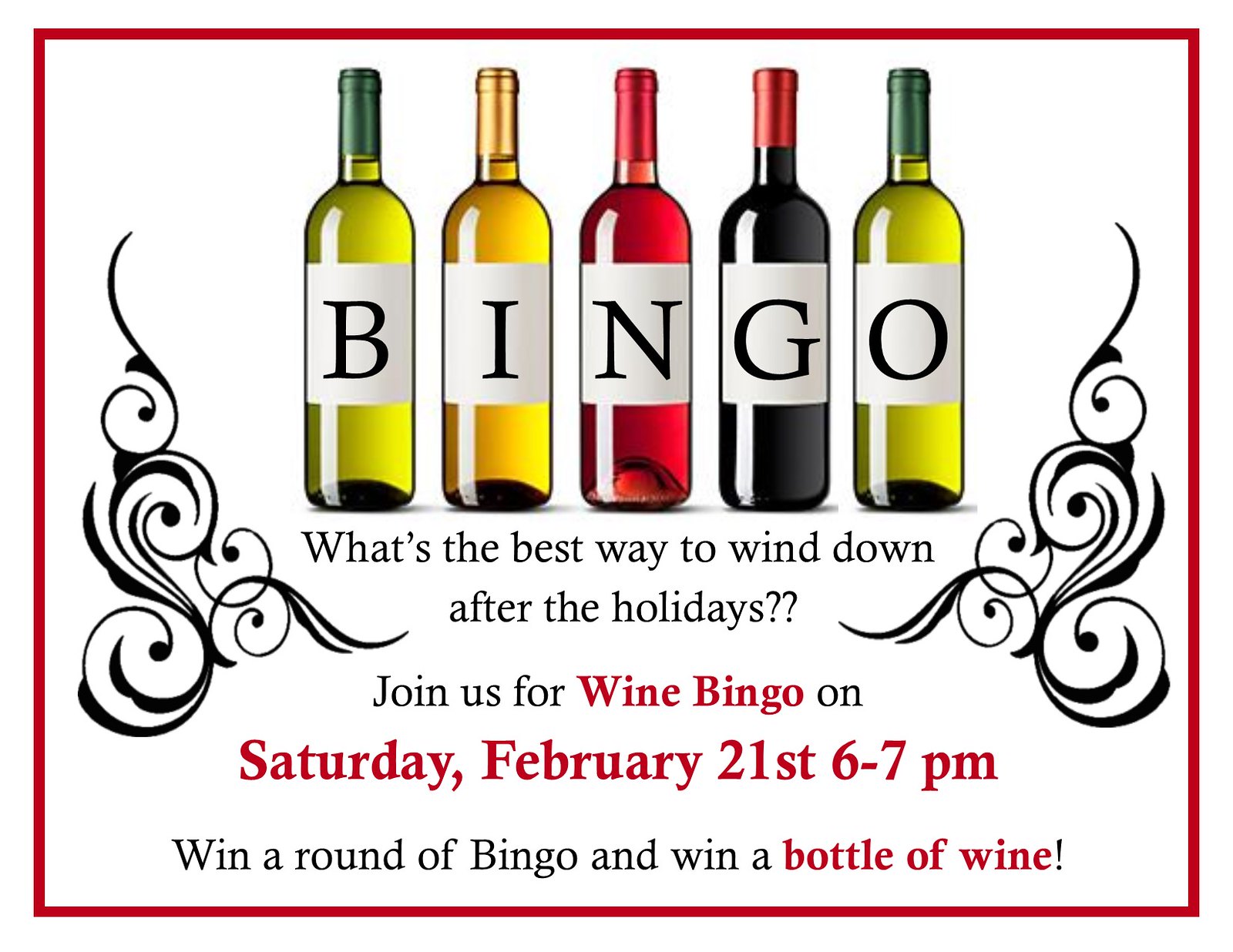The image is a festive advertisement featuring a white background with a thin red border, surrounded by decorative black swirls. At the top, five wine bottles are arranged in a line, colored respectively in green, yellow, red, black, and green. Each bottle has a label that together spells out "BINGO" in black lettering. Below the bottles, in black text, the caption reads, "What's the best way to wind down after the holidays?? Join us for wine bingo." The phrase "wine bingo" is highlighted in red. Following that, in large red font, it announces, "Saturday, February 21st, 6-7pm." At the bottom, it states, "Win a round of bingo and win a bottle of wine," with "bottle of wine" also highlighted in red and an exclamation point in black.